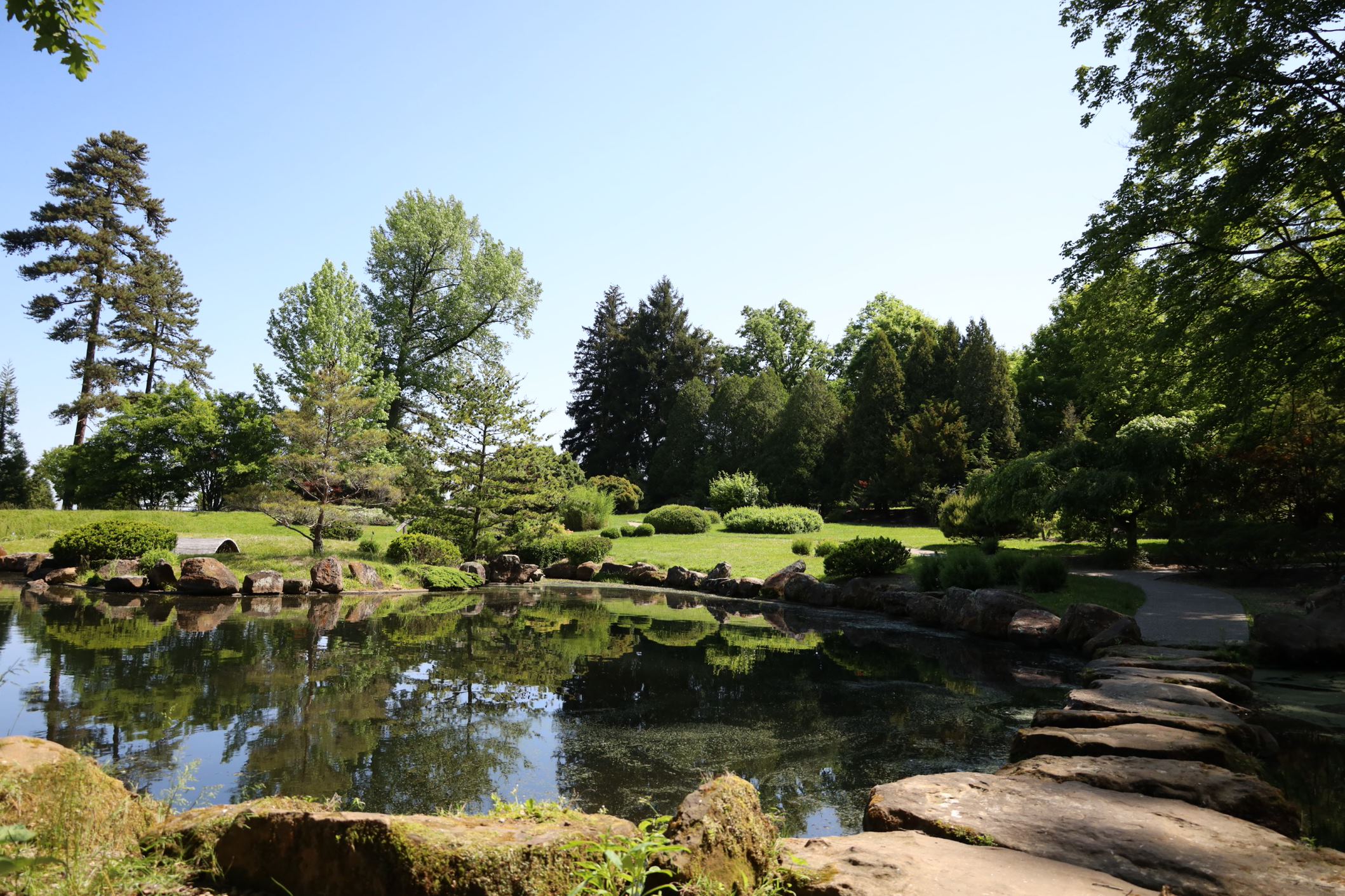A picturesque scene in nature showcasing a beautifully manicured landscape, reminiscent of a pristine golf course. A serene pond with a greenish hue is adorned with patches of moss and algae, reflecting the distant varieties of lush, green trees. A rock-covered path made of brown stones gracefully arches over the pond, leading to a neatly maintained sidewalk area. The vibrant, verdant grass and meticulously trimmed bushes contribute to the tranquil ambiance. Above, a clear blue sky stretches out, with the sun softly illuminating the open grassy fields, enhancing the natural beauty of the scene.